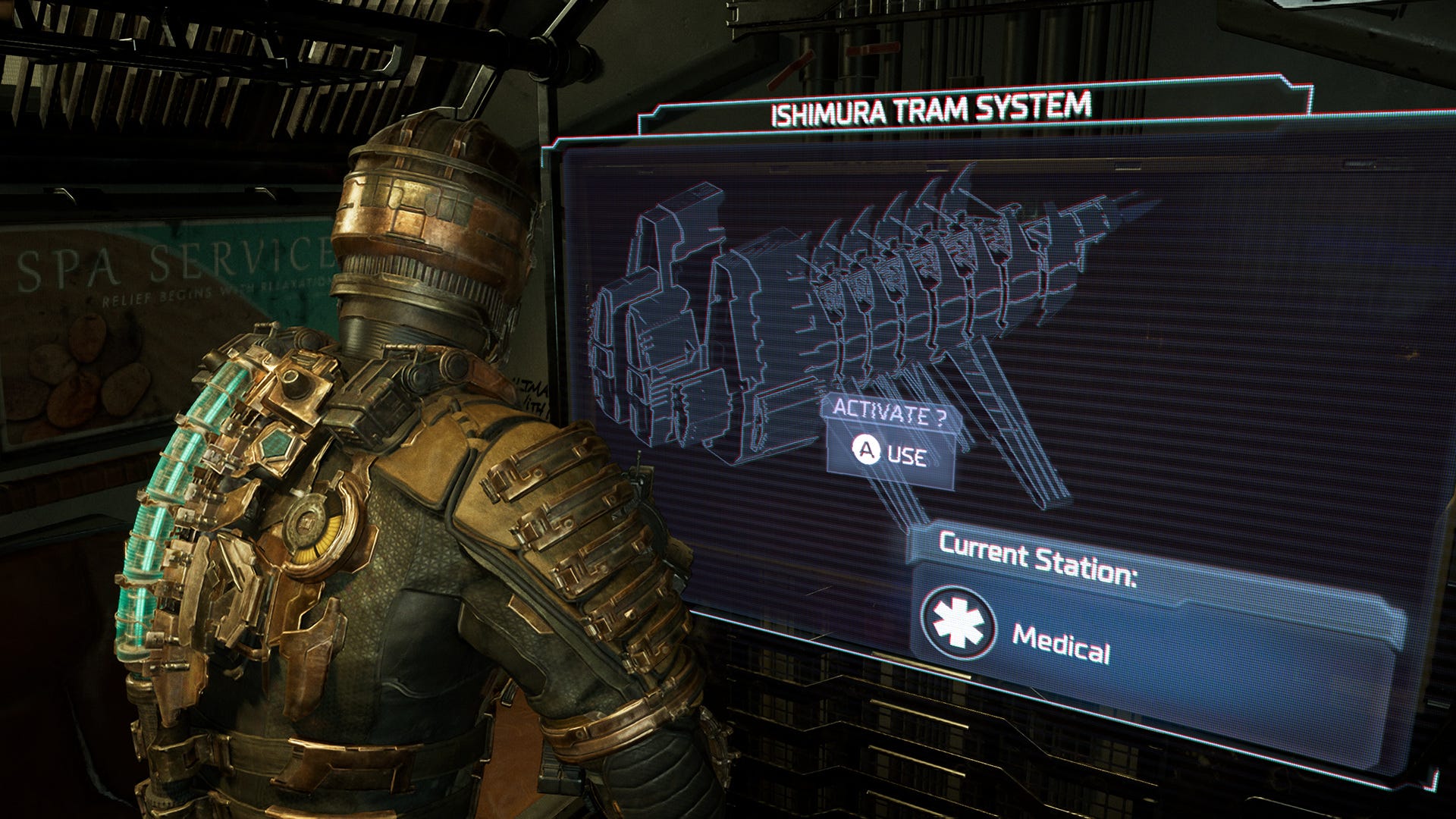In this detailed image, likely from a science fiction video game, we see a high-tech setting featuring a large touchscreen display. This display is titled "Ishimura Tram System" and shows a detailed diagram of what appears to be a tram or possibly a spaceship, with railings and controls included in the design. The screen also has the options "Activate?" and "Use," and indicates "Current Station: Medical" in blue and white text.

In the foreground, there is a figure that appears to be a soldier or robotic entity, heavily armored in a combination of bronze, green, and grayish-black colors. This character has a distinct, bronze-colored helmet or head and a pack on their back adorned with green lights, resembling a spine. The figure is fully mechanized, suggesting either advanced armor or a robotic form.

The background reveals a dark setting with green and brown hues, including walls with railings and grills. On the left side of the image, there is a shadowy advertisement that reads "Power Service. Relief begins with relaxation," suggesting a business ad within the game environment. The overall atmosphere is immersive and high-tech, emphasizing the intricate design and functionality of in-game elements and characters.